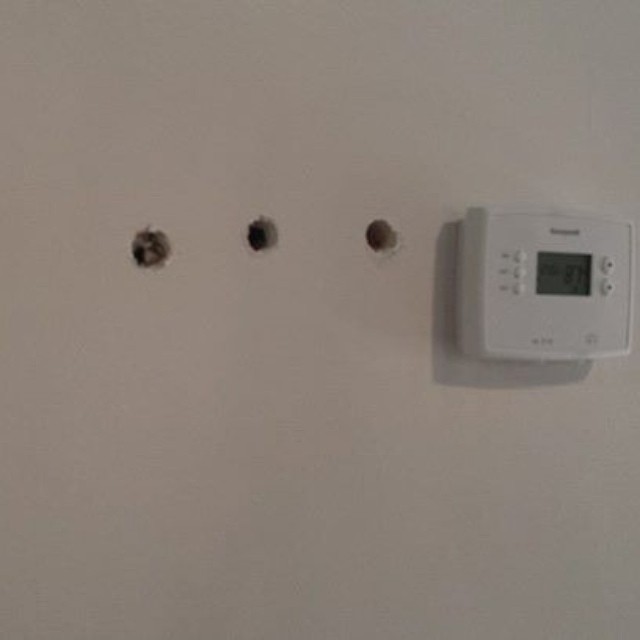In this dimly lit and slightly blurry image, an off-white wall is depicted, showcasing three irregularly spaced holes. These holes are not aligned either horizontally or vertically, creating a haphazard pattern on the wall. The largest hole appears to have remnants of white plaster protruding from it, with possibly a wire visible as well. The wall is observed from an oblique angle, adding to the imperfect perspective of the scene.

Adjacent to the holes, on the right side of the image, a Honeywell thermostat is mounted on the wall. The digital display on the thermostat clearly reads "10," while the remaining text is illegible. The device features three control buttons on the left side of the display, and up and down buttons on the right side. Beneath the display, there are two additional icons pointing towards two toggle buttons at the bottom of the unit. The multiple holes in the wall suggest that the thermostat may have been relocated several times, or perhaps different thermostats were installed in succession, each requiring a new placement.